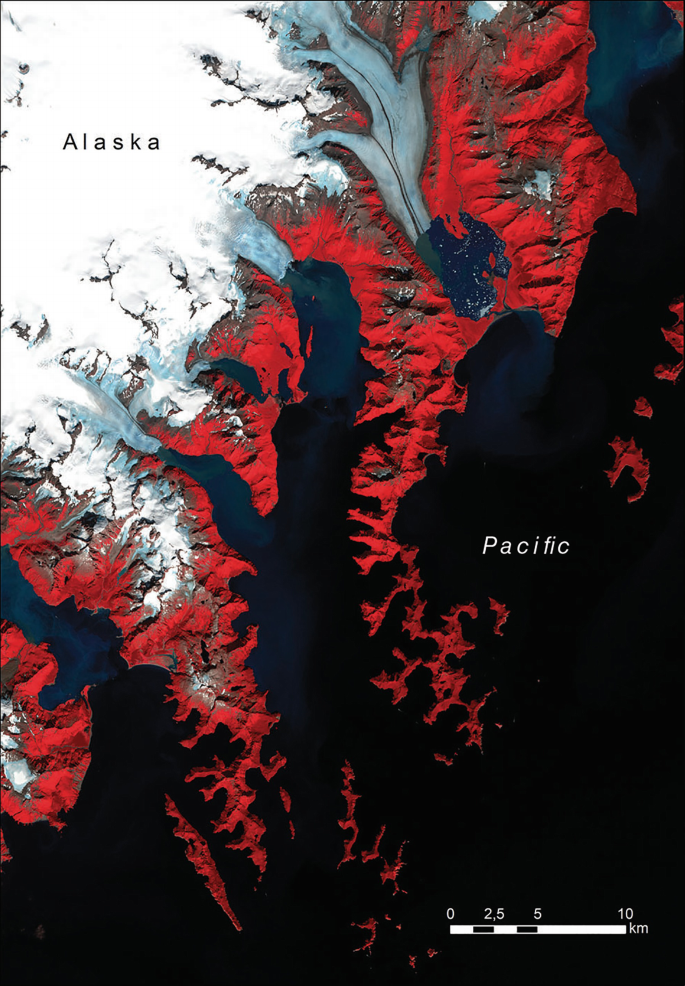This image is a detailed and color-enhanced digital map or satellite photograph focusing on the southern coastline of Alaska and the adjacent Pacific Ocean. The map vividly distinguishes various regions through color-coding: mainland Alaska, covered mostly in white likely due to snow, is contrasted with its coastal areas in dark red. Notable geographical features include peninsulas extending from the mainland and clusters of islands, alongside waterways that connect to the ocean. The Pacific Ocean is marked with a dark overlay and labeled 'Pacific.' In the bottom right corner, a white distance scale in kilometers (with denominations of 0, 2.5, 5, and 10) provides a measure of the area's extent, which spans roughly 100 kilometers by 200 kilometers. The map includes labels for Alaska and the Pacific, aiding in geographical orientation.